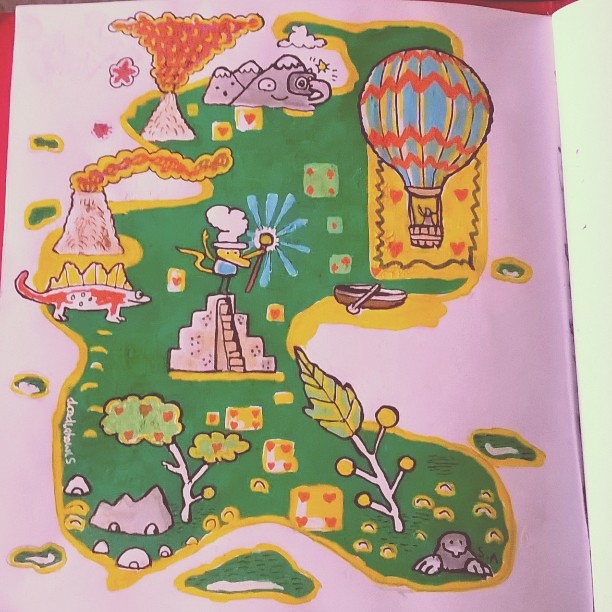The illustration depicts a vibrant and whimsical map of an island, reminiscent of those found in children's picture books. The island is lush and green, bordered by a bright yellow shoreline. In the top left corner, an erupting volcano sends a dramatic plume of fire skyward, while just below it, a larger volcano spews a long, thin stream of lava toward the right. Centrally located on the map is an imposing Aztec-style pyramid, crowned by a mysterious creature. The creature wields a staff in its right hand, which is topped with a glowing blue aura surrounding an amber or yellow bead. To the right, a large hot air balloon with an intricate pattern of blue, red, and yellow hues floats gently. In the bottom right corner, a curious mole is seen emerging from the ground, adding a touch of earthy charm to the fantastical scene.